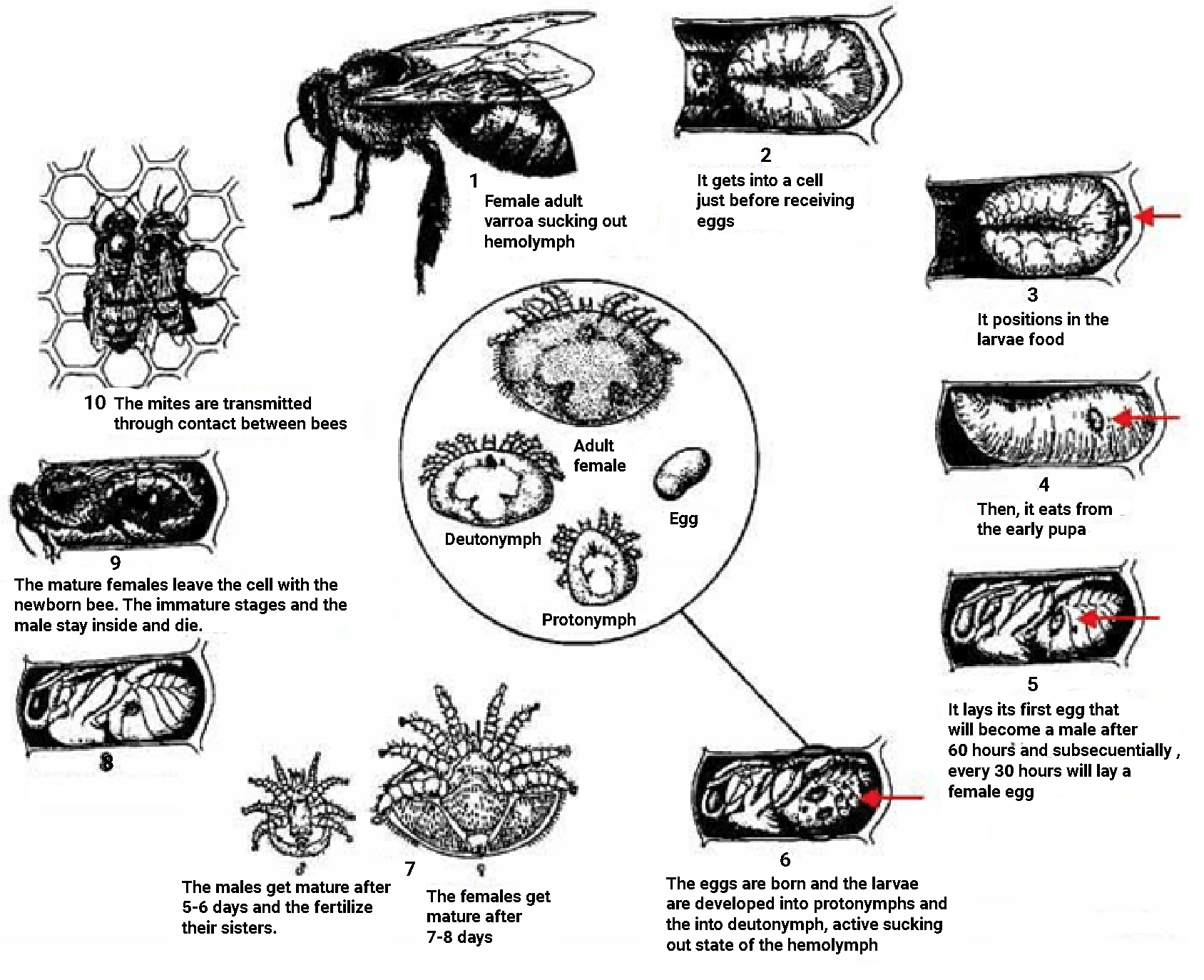The infographic is a detailed black and white scientific diagram illustrating the reproductive cycle of the Varroa mite, a parasite of bees. The diagram is structured in a circular format, with stages labeled from one to ten. Each stage provides insights into the life cycle of the mite, complemented with images and descriptions.

At stage one, the illustration depicts an adult female Varroa mite, characterized by its oval body and hairy legs, actively sucking out the hemolymph of a bee. Stage two shows the mite entering a cell just before the bee larvae receive their food. At stage three, the mite positions itself within the larval food, laying its first egg which will develop into a male after approximately 60 hours. Subsequently, every 30 hours, it lays a female egg. 

Stage four details the formation of a pupa, while stage five describes the initial development of the male mite. By stage six, the eggs have hatched, and the larvae are developing into protonymphs and then into deutonymphs, actively feeding on the host hemolymph.

Stage seven reveals that the female mites become fully mature after seven to eight days, while males mature within five to six days and then fertilize their sisters. In stage eight, illustrated is a nearly full-sized bee and the mature female mites leaving the cell with the newborn bee. The immature mites and males remain in the cell and eventually die.

Stage nine and ten illustrate the final steps of mite transmission, showing the newly emerged mites on a honeycomb, ready to infest other bees through contact. The center of the diagram also highlights the developmental stages of the mite, from eggs to deutonymphs. Each illustrated stage complements the text-heavy, scientific explanation, providing a comprehensive understanding of the Varroa mite's life cycle and its impact on bees.